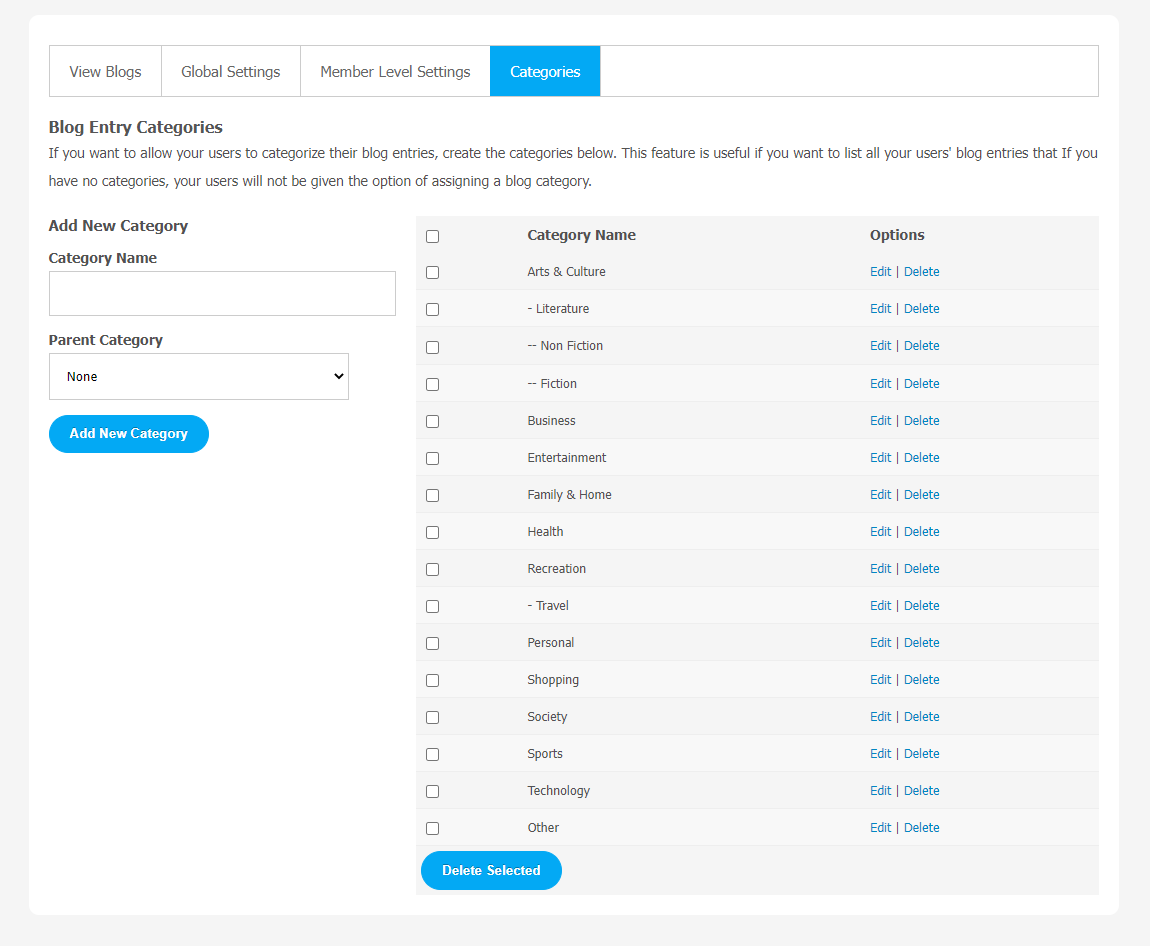The interface displays a clean, organized layout with a light gray border enclosing the top section featuring a white background. The top navigation includes several menu options in gray text: "View Blogs," "Global Settings," "Member Level Settings," and "Categories." The "Categories" option is distinctly highlighted in a bright blue box with white text, indicating it is currently selected. 

Below the menu, a bold black heading reads "Blog Entry Categories." This is followed by an explanatory note in small gray font: "If you want to allow your users to categorize their blog entries, create the categories below. This feature is useful if you want to list all of your users' blog entries. If you have no categories, your users will not be given the option of assigning a blog category."

Further down, the interface prompts users to "Add New Category" in bold letters. Under this, it asks for a "Category Name" with an editable rectangular field bordered in light gray for input. Next, a smaller bold label "Parent Category" accompanies a dropdown menu, with "None" being the default selection.

To confirm and create a new category, there is an oval button with a bright blue background and bold white text that says "Add New Category."

On the right side, a table is presented with alternating row colors for clarity. The first two rows are a consistent light medium gray, followed by a patterned alternation between light and medium gray rows.